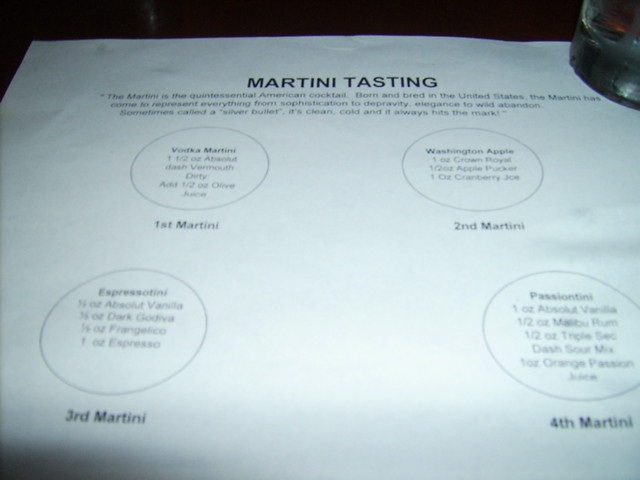The image reveals a close-up of a white piece of paper titled "Martini Tasting," placed on a brown wooden surface. The top-left and top of the image feature a black background, while the upper right corner partially shows a frosted glass with what appears to be a red pale ale. 

The paper prominently displays "Martini Tasting" in bold black capital letters. Beneath the title, there is a short, somewhat illegible paragraph that discusses the iconic status of martinis in American culture, touching on their variety and appeal. The main focus of the paper is four labeled circles, arranged in two rows. Each circle indicates a different type of martini along with its ingredients. The four types listed are: 

1. Vodka Martini – includes ingredients difficult to decipher but mentions Absolut and vermouth.
2. Washington Apple – partially readable, mentioning Crown Royale and cranberry juice.
3. Espresso Trini – ingredients include Absolut vodka, dark Godiva, and espresso.
4. Passion Tini – lists Absolut vodka, Malibu rum, triple sec, and orange passion juice.

The detailed descriptions within the circles provide recipes, although some parts are too blurry to make out clearly. The setting appears to be indoors.